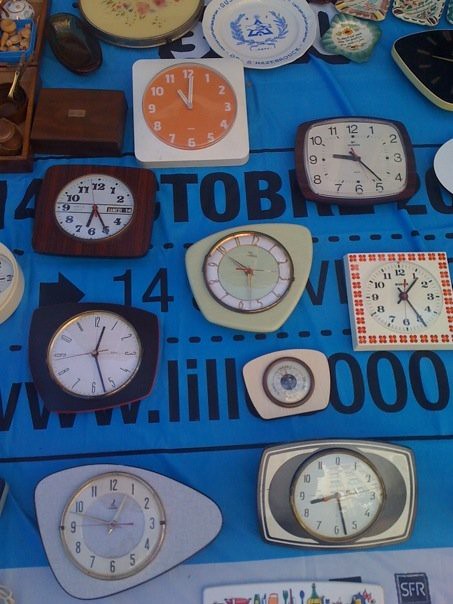This photograph captures a collection of vintage clocks meticulously arranged on a light blue cloth adorned with indistinct black writing, including parts of an email address. The clocks, numbering between 12 and 15, showcase a variety of shapes and sizes, typical of mid-20th century design, including circular, square, rectangular with curved edges, and uniquely oblong forms. Predominantly intended for bedside use, their aged appearance suggests they are over 50 years old, with most featuring conventional numbers except for one, which resembles a compass. A few clocks are highlighted by wood exteriors. Surrounding these timepieces are additional items transitioning at the top of the image into what appear to be ceramic dishes, possibly ashtrays, and blue-floral inlaid white porcelain pieces, hinting that this setup might be part of a flea market or antique dealership display. The background is barely visible due to the dense arrangement of the clocks, complementing the vintage ambiance of the scene.